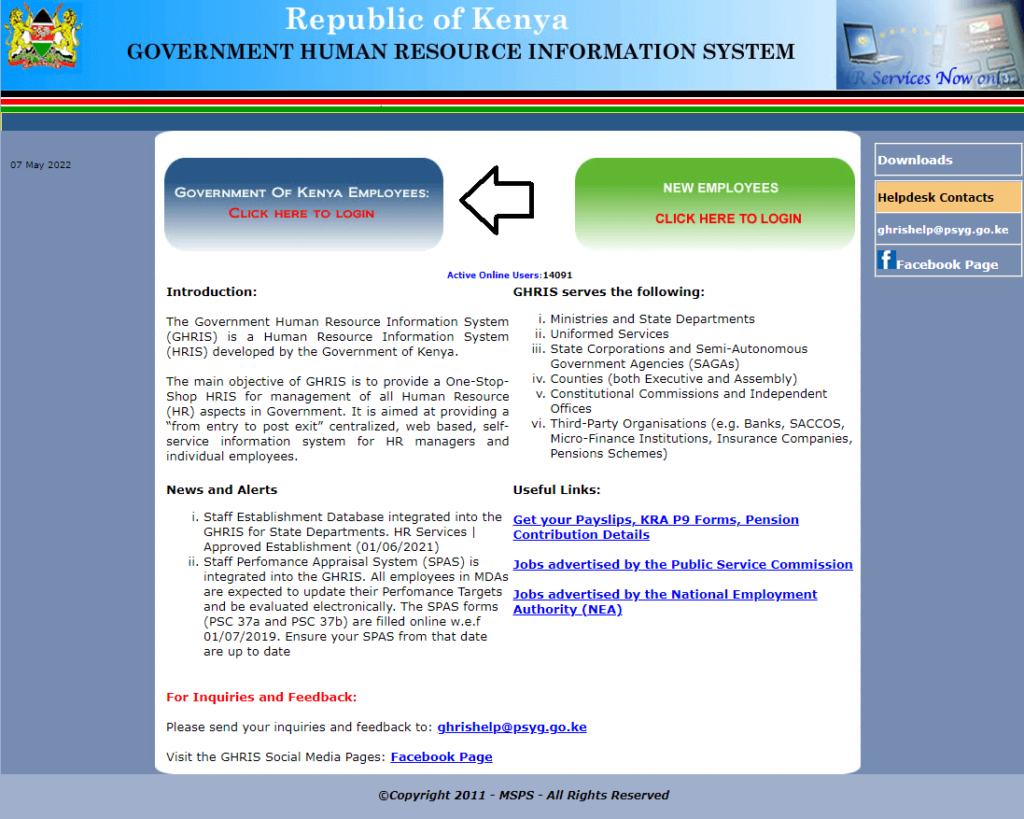**Screenshot of the Republic of Kenya Government Human Resource Information System (GHRIS) Website**

The screenshot captures the homepage of the Government Human Resource Information System (GHRIS) website. At the top, a blue banner features the official logo on the left, reading "Republic of Kenya, Government Human Resource Information System". On the top right, there is an image of a laptop with the text "PR Services Now Online".

Beneath the banner are thin horizontal bars in the national colors: black, red, and green. To the left side, a gray section displays the date "07 May 2022".

The central portion of the page is predominantly white, featuring two prominent buttons for user login. A blue rectangle labeled "Government of Kenya Employees. Click here to log in." includes an arrow pointing left. Below it, there is a green rectangle labeled "New Employees. Click here to log in."

Directly beneath these buttons, text indicates that there are "Active Online Users: 14091". The main body of the screen provides a detailed introduction to GHRIS, outlining its purpose and objectives. GHRIS is described as a centralized, web-based, self-service HR information system developed by the Government of Kenya to manage all human resource (HR) aspects within government organizations. The platform supports various entities, including ministries, state departments, uniformed services, state corporations, semi-autonomous government agencies (SAGAs), county governments, constitutional commissions, independent offices, and third-party organizations.

In the “News and Alerts” section, the following updates are detailed:
1. The staff establishment database has been integrated into GHRIS for state departments with an approved establishment date of 1-6-2021.
2. The Staff Performance Appraisal System (SPAS) is integrated with GHRIS, requiring all employees and Ministries Departments and Agencies (MDAs) to update their performance targets and undergo electronic evaluations. Forms PSC 37A and PSC 37B are to be filled online with effect from 1-7-2019. 

For inquiries and feedback, users are directed to contact GHRIS help via email at ghrishelp@psyg.go.ke. Users are also encouraged to visit the GHRIS social media pages for more information.

The page footer includes useful links for accessing payslips, KRA P-9 forms, pension contribution details, and advertised jobs by the Public Service Commission and the National Employment Authority (NEA). Additionally, there are options for downloads and helpdesk contacts, reiterating the GHRIS help email and Facebook page.

The website carries a copyright statement of © 2011 MSPS, all rights reserved.